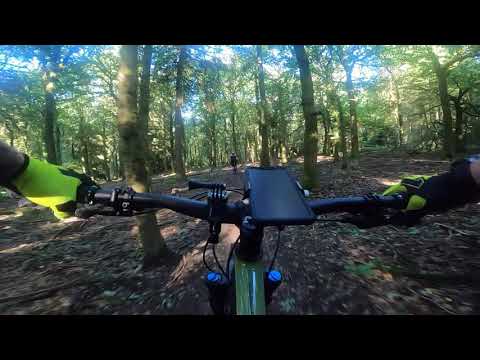The image is a horizontally aligned, rectangular picture with thick black borders at the top and bottom. It captures the scene of a forest area with numerous tall, somewhat curved tree trunks and green leaves forming a canopy overhead. Between the leaves at the top, rays of yellow sunlight filter through, revealing patches of a bright, blue and white sky, indicating it is daytime. 

In the foreground, a mountain bike's front end is prominently visible. The rider's hands, clad in neon yellow and black gloves, grip the handlebars, which are equipped with a small slot holding a cell phone, likely for navigation. The gear shifter is also visible, along with a metallic part of the bike that appears to be either brown or green, though the exact color is difficult to discern.

The ground is a mix of dirt, leaves, and twigs, creating a natural, rugged path. Another individual, possibly also on a bike, is faintly visible further down the trail, dressed in black. The overall scene evokes the adventure of a sunny day bike ride through a serene, sun-dappled forest.